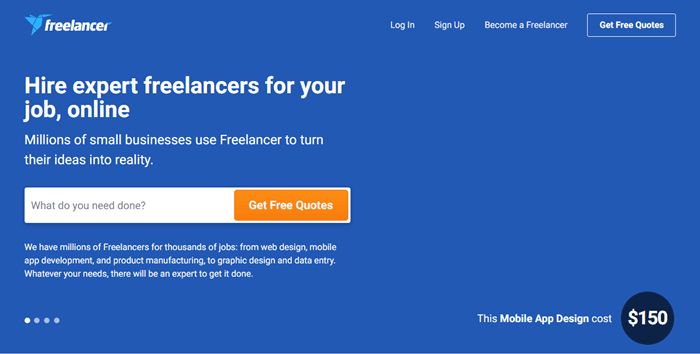This section depicts a dark blue webpage interface. In the top left corner, a cyan blue bird icon is situated next to the white text "freelancer," highlighted by a capitalized "R" in blue. On the right hand side, user options such as "Log In" and "Sign Up" are listed, followed by "Become a Freelancer." A white-bordered button with bold white text states "Get Free Quotes."

Below, in bold white lettering, the phrase "Hire Expert Freelancers for Your Job, Online" stands prominent. A subsequent line in thin white text indicates, "Millions of small businesses use Freelancer to turn their ideas into reality." Positioned below is a white rectangular input field with gray text asking, "What do you need done?"

To the right of this input field is an orange button with bold white text reading, "Get Free Quotes." Underneath, white text informs, "We have millions of freelancers for thousands of jobs, from web design, mobile app development, and product manufacturing, to graphic design and data entry. Whatever your needs, there will be an expert to get it done."

At the bottom, four ellipses are shown, with the first filled in white and the remaining three in a faded blue, matching the background. On the right-hand side, a section reads "This Mobile App Design Costs," with each word of "Mobile App Design" capitalized and in bold white text, whereas "This" and "Costs" are not bolded. A black circle is displayed showing the cost of web design as "$150."